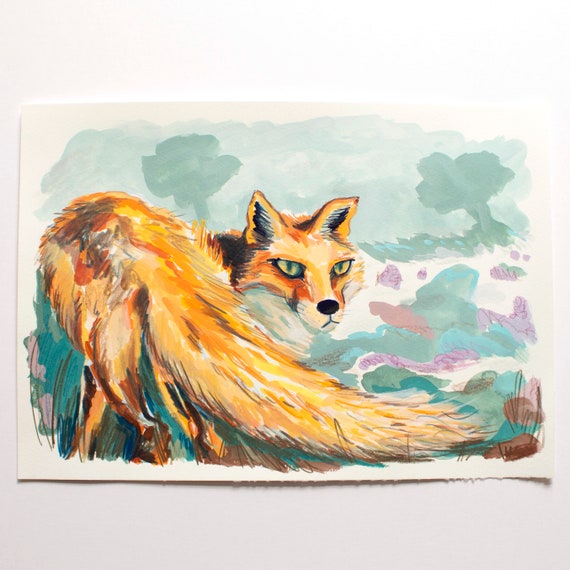This is a detailed and striking watercolor painting on a white canvas. The painting features a highly detailed red fox, positioned with its body facing away from the viewer while its head is turned back, directing its sharp, bright yellow eyes straight at the observer. The fox has a reddish-brown coat, with intricate brush strokes that effectively convey the texture of its fur, a black nose, and black-lipped mouth, and white markings on its cheeks that blend into the brownish-red color of its fur. Its ears show black shadows accentuated with white hair, enhancing the lifelike quality. A large, bushy tail obscures much of the fox's body. The expression on the fox's face is intensely focused, evoking a sense of irritation or displeasure. The background is an abstract mixture of blue, green, purple, red, and orange shapes, which seem to represent trees, flowers, and perhaps elements of the sky and ground, creating a vibrant yet somewhat chaotic setting. Blue and green hues suggest both grass and sky, while scattered purple specks add to the complexity of the scenery. The entire composition vividly captures the focus and the underlying tension in the fox's demeanor against a dynamic, colorful backdrop.